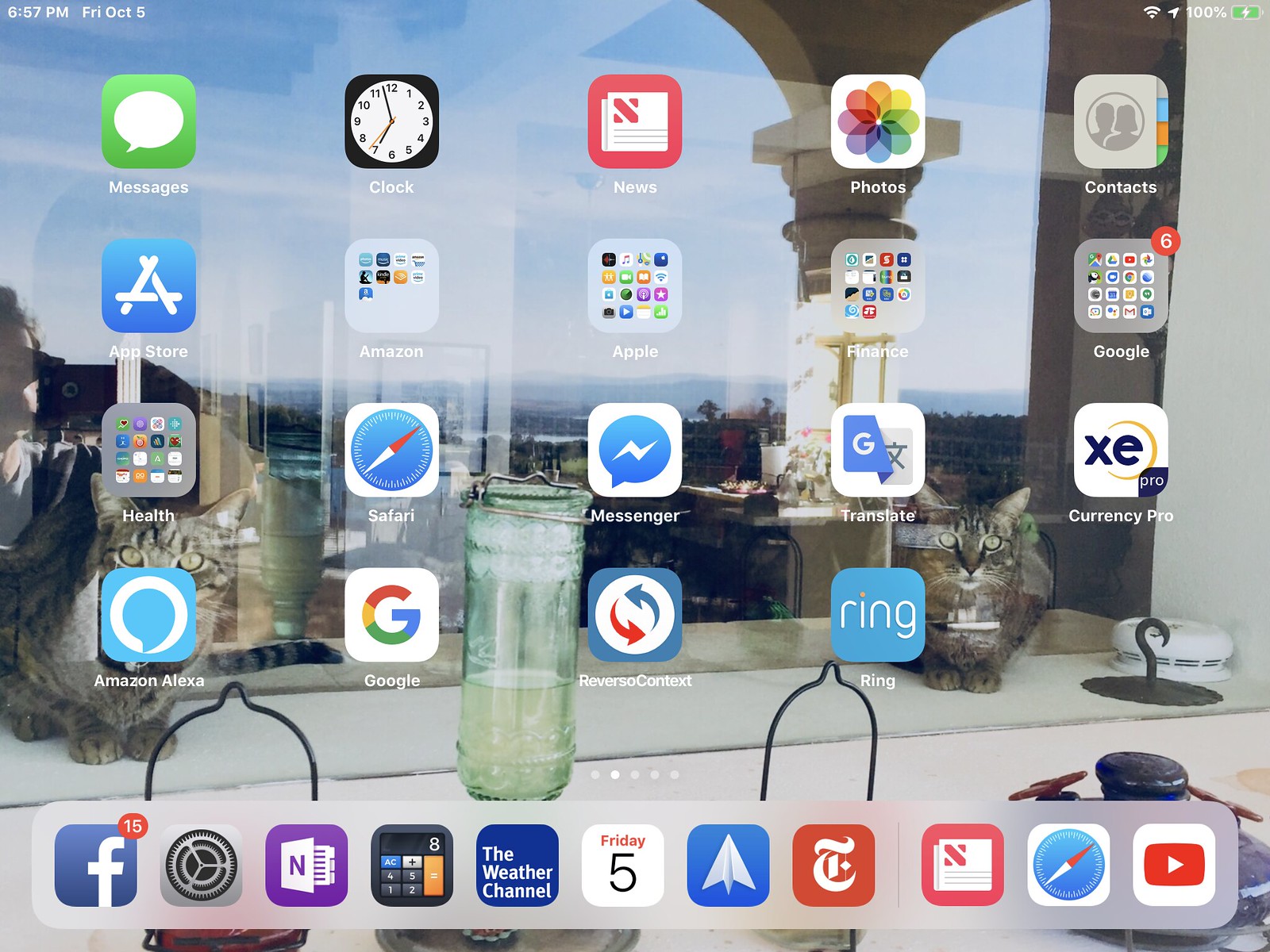This photograph captures a close-up view of someone's computer desktop screen. The background image features an outdoor scene with a vivid blue sky and a distant mountain range. The foreground shows a bit of the landscape, providing a serene and picturesque backdrop. Prominently displayed in the center of the wallpaper is a charming gray tabby cat.

The desktop is filled with a variety of icons, organized from top to bottom. The top row includes icons for Messenger, Clock, Google Photos, and Contacts. Below these, there's a folder labeled "Google Apps," followed by icons for the App Store and Safari browser. Additional icons include Facebook Messenger, Ring (the home security device), and Google. Toward the bottom of the screen, popular applications like Facebook, The Weather Channel, The New York Times, YouTube, and several others are visible. The array of icons indicates a well-used and organized desktop, set against a calming and visually pleasing backdrop.